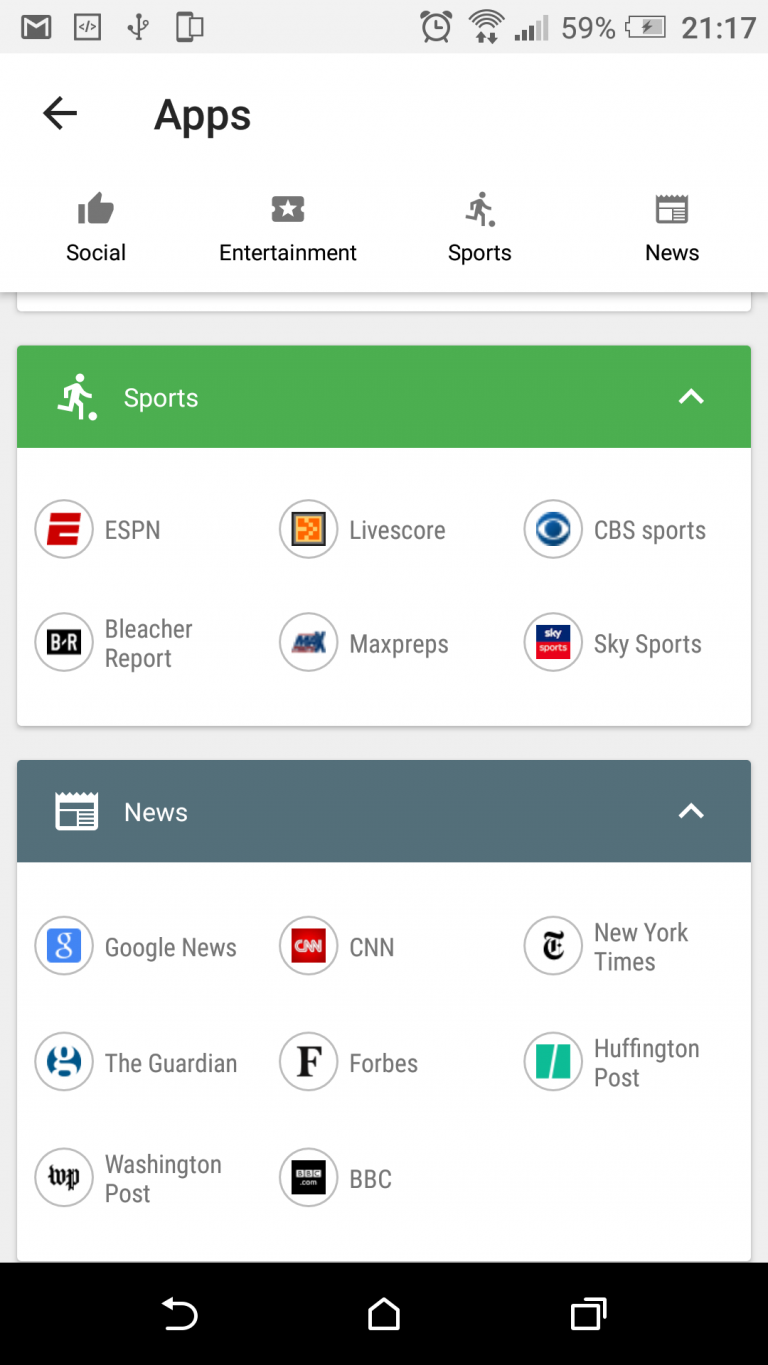Here is the cleaned-up and detailed caption for the described image:

---

The screenshot displays a mobile phone interface. At the very top, there's a left-pointing arrow labeled "Apps." Below that, the screen is divided into four tabs: "Social," "Entertainment," "Sports," and "News." The primary section in focus belongs to the "Sports" tab, indicated by a rectangular box with a green strip at the top featuring a stick figure icon of a person kicking a soccer ball.

In this section, there are six app icons, organized into two rows and three columns. The first row consists of icons for ESPN, LiveScore, and CBS Sports. The second row features icons for Bleacher Report, MaxPreps, and Sky Sports. 

Below the sports section is another rectangular box dedicated to the "News" tab. This section has a blue banner at the top with the word "News" written in white. It also includes an icon symbolizing a newspaper. Within this section, there are eight app icons arranged in three rows and three columns. The first row displays icons for Google News, CNN, and The New York Times. The second row includes icons for The Guardian, Forbes, and HuffPost.